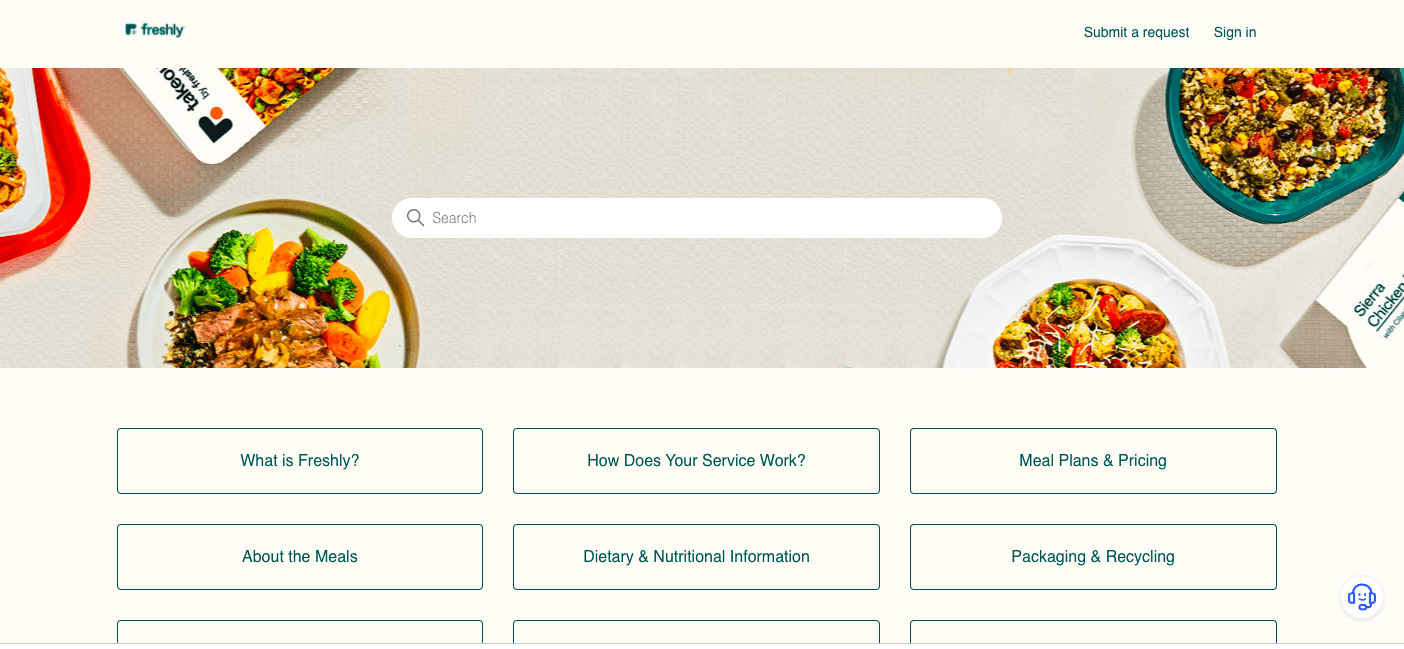The website interface prominently features the brand "Freshly" in the top left corner, while the top right corner houses options for "Submit a Request" and "Sign In." Immediately below these options is a large, full-width rectangular banner image showcasing various dishes. 

The banner includes:
- A white bowl filled with food.
- A green bowl containing another dish.
- On the far left, there's a partial view of a red-bordered white plate with food.
- Below this, a white plate displays an assortment of green, yellow, orange, and brown foods.
- To the far right, a second white plate is adorned with what appears to be green, red, and yellow ingredients, potentially including rice. 

Directly beneath this banner are several informative boxes arranged in rows:
1. "What is Freshly?"
2. "How Does Your Service Work?"
3. "Meal Plans and Pricing"
Completing the first two rows:
4. "About the Meals"
5. "Dietary and Nutritional Information"
6. "Packaging and Recycling"

Although three more boxes are partially visible, their contents are obscured. To the right of these boxes is a small headphone icon, likely indicating customer support.